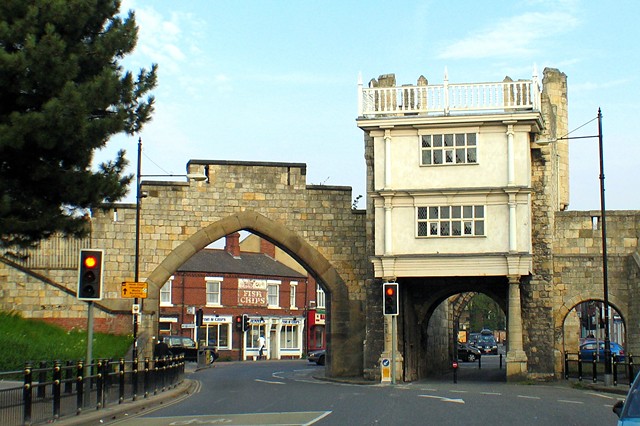This detailed photograph captures a charming town intersection, possibly in Great Britain, characterized by its brick architecture and medieval appearance. Dominating the scene is a traffic circle with traffic lights, both glowing red. The intersection is framed by a grand walled entrance, made up of tan, light brown stone bricks, featuring a large central archway alongside two smaller semicircular arches to the right, commonly seen in European towns.

Beyond the entrance, a brick building prominently displays a sign for "Fish and Chips," hinting at the town's British locale. The building is painted red, complementing the old-world charm of the town. Above one of the smaller arches, there appears to be an old guard post or sentry station, with small windows that once served as lookout points.

Visible through the arches are parked cars, suggesting a bustling yet quaint village atmosphere. To the left of the intersection, a large tree stands beside the traffic light, adding a touch of greenery to the scene. The sky above is a serene blue, adorned with wispy clouds, enhancing the picturesque quality of this European town.